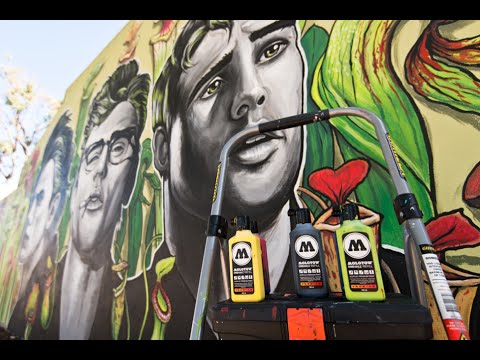The mural is a striking black-and-white portrait of three lifelike Caucasian men in their early 20s, prominently featuring the man in the middle who wears glasses while the other two do not. All three are depicted from the shoulders up, showcasing their full heads of hair. The vibrant background contrasts sharply with the monochromatic figures, adorned with lush green foliage and red floral elements. Situated outdoors, likely along the side of a highway or road, the mural is accompanied by a small step ladder and three paint tubes—yellow, gray, and light green—indicating the tools used by the artist. Positioned near some trees and greenery, the mural adorns an exterior wall, marked by a large M emblem, adding a touch of color to the otherwise grayscale depiction.